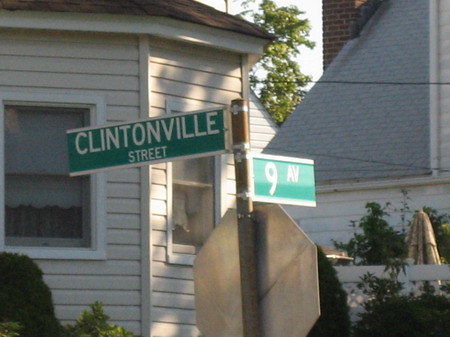The image captures a street corner, prominently featuring the back of a stop sign at its center. The pole supporting the stop sign also holds two green street signs. The top sign, facing the camera, reads "Clintonville Street" in white font, with "Clintonville" displayed larger and above "Street." Below it, a second green sign is angled slightly to the right, displaying the number "9" in white font, with an abbreviation "A-V" located at the upper right-hand side of the sign.